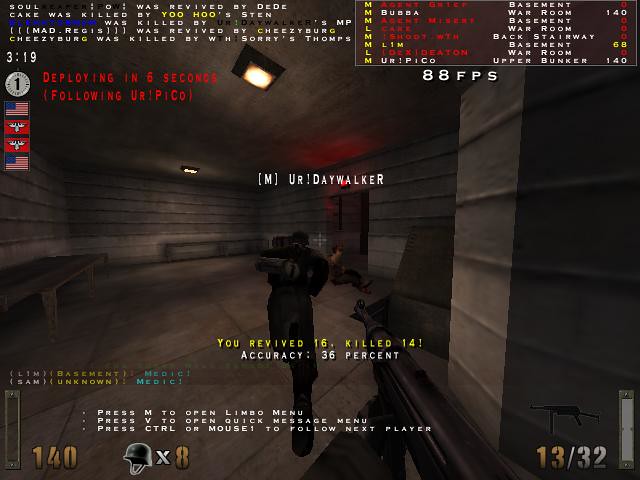This image is a still from a dark and gritty first-person shooter video game. The player character, seen from a first-person perspective, is dressed in dark clothing, adding to the shadowy, tense atmosphere. In the player's hands, a gun extends outward, indicating readiness for confrontation. The setting appears to be an ominous concrete room, likely a fortress or bunker, with walls that suggest confinement and danger. The environment is further characterized by text overlays scattered around the screen, providing critical in-game statistics. In the center, prominent text reads: "M, Yuri Daywalker. You revived 16, killed 14. Accuracy: 36%." This text likely indicates the performance metrics of the player or another in-game character. Overall, this detailed snapshot captures the essence of a suspenseful and action-packed moment within the game.